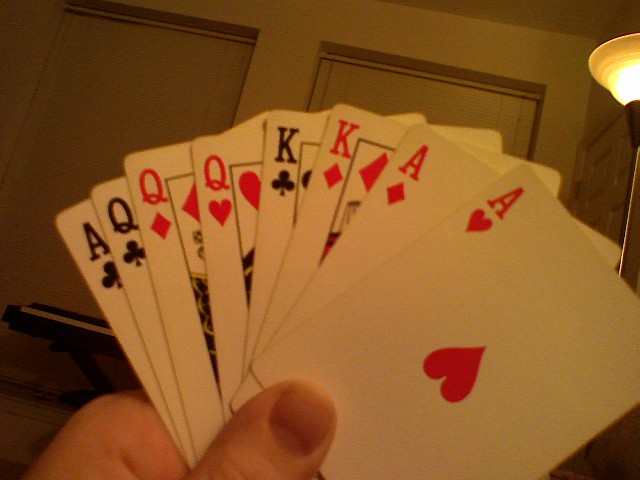The image captures an indoor setting, with a prominent ceiling or wall-mounted light fixture located in the upper right-hand corner. The light has a muted glass shade and emanates from a base at the bottom, illuminating upwards, although it is unclear if the light continues down the wall. The ceiling features wooden panels that are painted a beige color.

The focal point of the image is a left hand holding a fan of eight playing cards. The thumb, sporting a short, clean-cut nail and well-maintained cuticle, is visible. The specific cards held, from left to right, are: Ace of Clubs, Queen of Clubs, Queen of Diamonds, Queen of Hearts, King of Clubs, King of Diamonds, Ace of Diamonds, and Ace of Hearts. The cards are plain with no intricate designs; notably, the Ace of Hearts features just a heart symbol in the center.

In the background, just behind the thumb area of the hand, there is a black element with a white bar across it. The overall composition centers on the hand of cards, emphasizing the details of the cards and the subtle elements of the indoor setting.